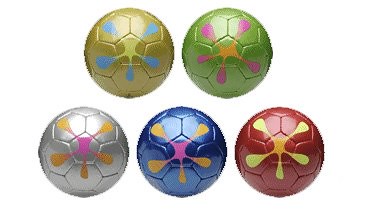This detailed image features five glossy, multi-colored soccer balls set against a very white background. Arranged in a small pyramid formation, two balls are positioned at the top followed by three directly below. Each ball is uniquely colored—silver, blue, orange, green, and yellow—and showcases a distinctive pattern of hexagons that mimic the design of traditional soccer balls.

Each ball is adorned with a star-like dot pattern: the yellow ball has blue spokes and a yellow center, the orange ball features yellow spokes with an orange center, the green ball has pink spokes with an orange center, the blue ball shows orange spokes with a pink center, and the silver ball is characterized by orange spokes with a pink center.

The balls do not touch each other and, although similar in design, each one’s color scheme and dot arrangement make them unique. Despite appearing against a void-like white backdrop, they stand out due to their shiny, glossy surfaces and the intricate colorful details.

Together, they collectively create a visually striking arrangement, reminiscent of a pyramid, yet uniquely individual in their vivid colors and star-like patterns.